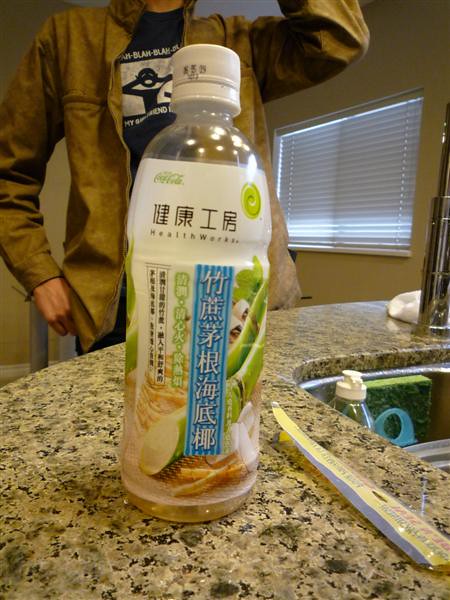The image depicts the interior of an apartment or house. On the right side of the frame, beige-colored walls are visible, along with a rectangular window adorned with white blinds. In the bottom right-hand corner, there's a sink with a silver faucet, where a portion of the sink contains a gray object that might be a dish. Nearby, a bottle of dish soap with a white top and clear body is present, alongside a sponge holder holding a sponge that's green on top and yellow-green on the bottom. The countertop is made of a marble-like material, exhibiting a blend of brown and black colors. Additionally, a water bottle with Asian characters written in white, green, and black lettering sits on the surface. The bottle has a white cap and features a green illustration, possibly of sugar cane. In the background, a person wearing a black jacket and a black-and-white t-shirt is partially visible.